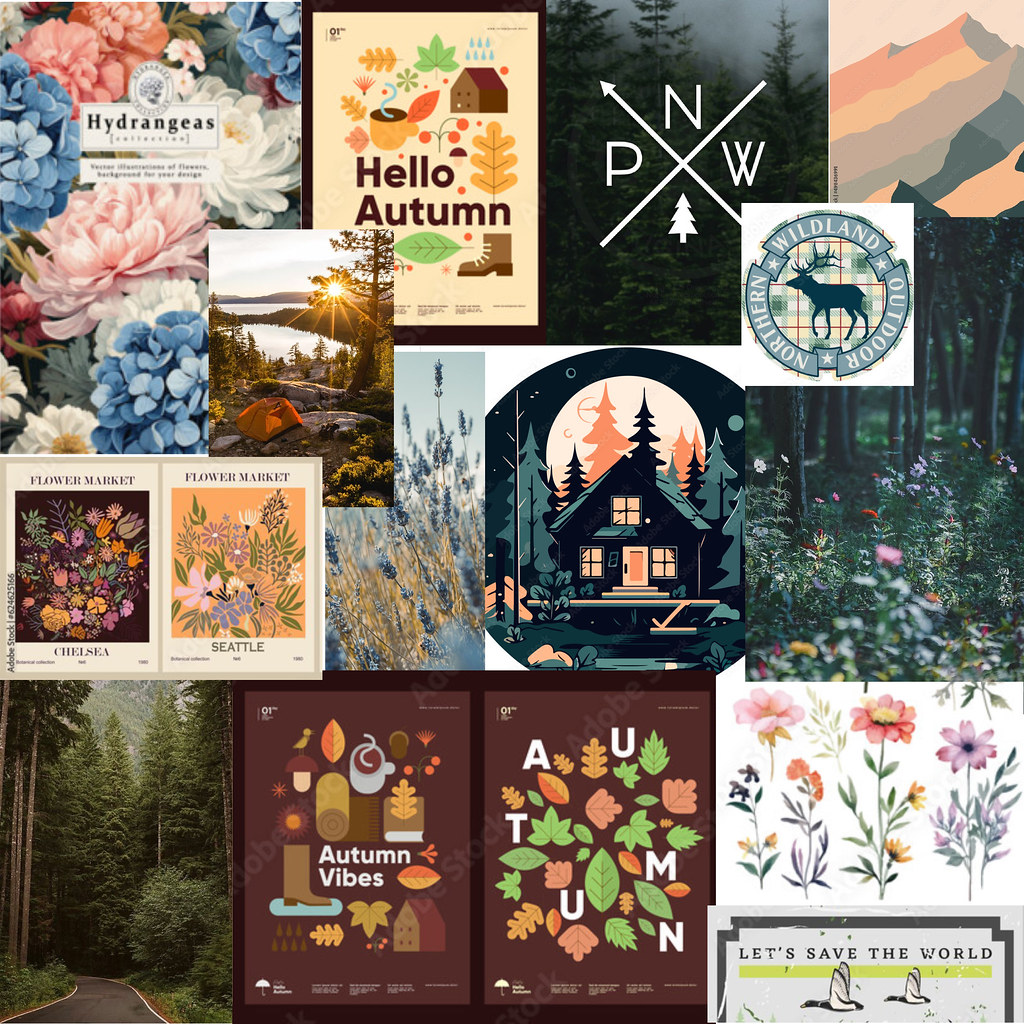This intricate collage captures the essence of both autumn and spring, filling the image with a spectrum of seasonal vibes. Dominating the top left corner, vibrant hydrangeas in pink, white, and blue hues are juxtaposed with a card reading "Hello Autumn," adorned with fall leaves, a cup of coffee, and hiking boots. Adjacent to it, a cross marked with "P, N, W" encapsulates the Pacific Northwest spirit with pine trees and watercolored mountains. A "Northern Wildland Outdoors" emblem features an elk amidst a scenic meadow. Various layers of the collage bring to life the beauty of a country road winding through cedar and pine trees, a rustic logging house, and a camping site set against the backdrop of a tranquil lake, trees, and distant mountains, bathed in the setting sun.

Peppered throughout the collage are nods to flower markets, including signs from Chelsea and Seattle, showcasing an array of blossoms. There are also multiple references to autumn, with overlapping symbols of fall leaves, hot cocoa, and encouraging phrases like "Let's Save the World." Spring elements peek through with pastel flowers adding lightness and color contrast. The lower left corner captures a serene country road lined with towering trees, while other spots feature a remote tent setup, reinforcing the collage’s outdoor and nature themes, transforming the image into a complex tapestry celebrating the cyclical beauty of nature.